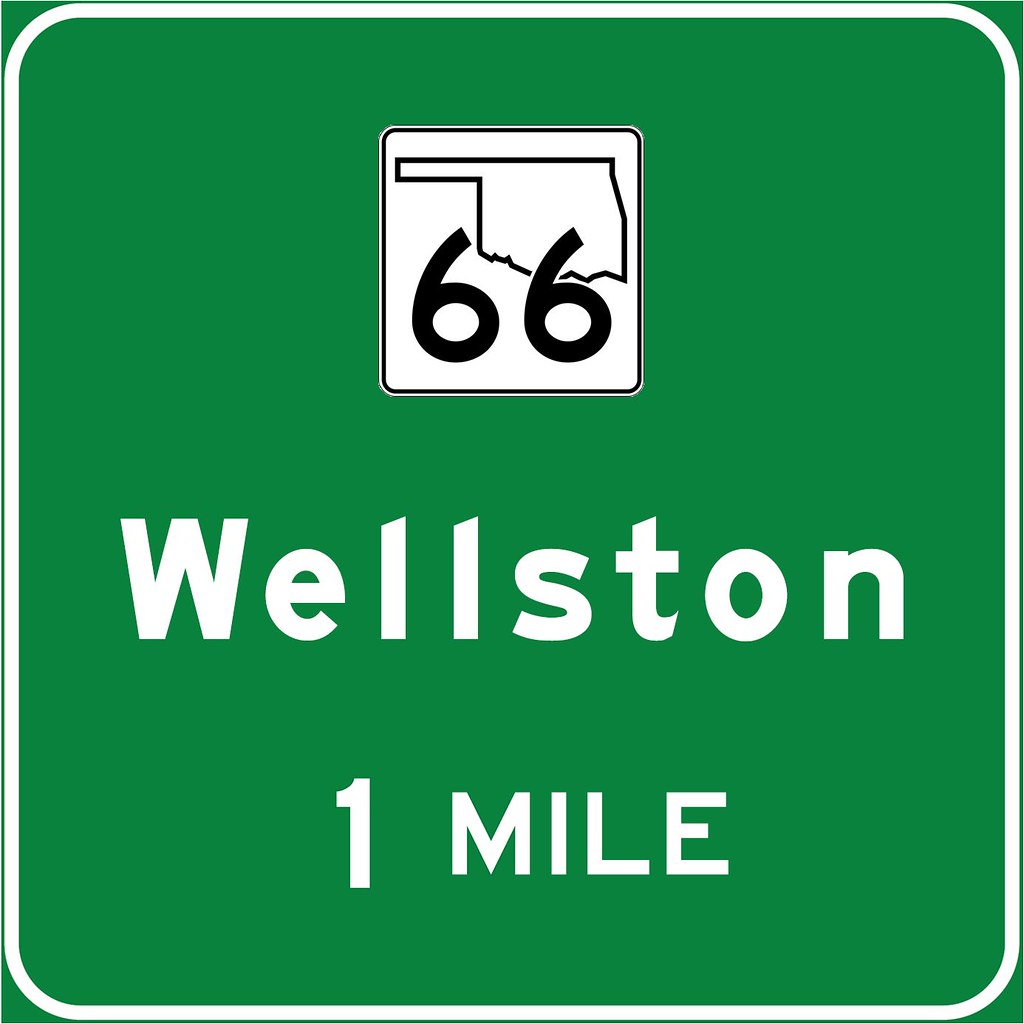This is a full-color image of a road sign. The main background of the sign is green with a slightly lighter white border that curves at the edges, resulting in small green triangles at each corner. Dominating the top section of the sign is a square with a black outline. Inside this square is a symbol resembling a leftward-facing hand, which might be an abstract representation of a U.S. state, though its exact identity is unclear. Directly below this symbol, in bold black print, are the numerals "66."

Further down on the green background, large yellow text spells out "Wellstone," with noticeable spacing between each letter and only the initial "W" capitalized. Beneath "Wellstone," the phrase "One Mile" is written in smaller yellow letters, placed more closely together than those above. The overall imagery is crisp and clear, and no additional elements are present in the image.